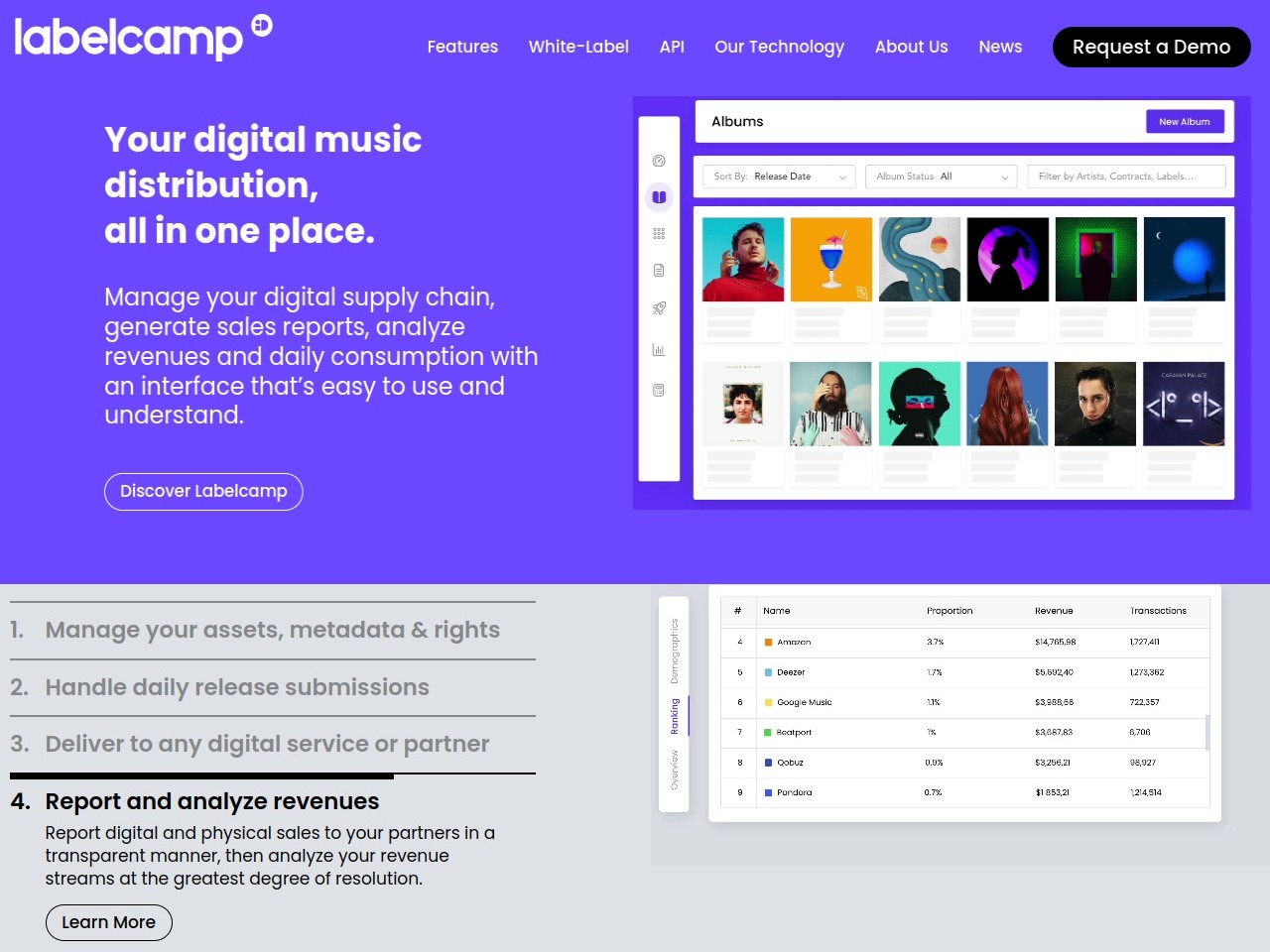The image features a user interface with a light purple header at the top displaying the text "Label Camp." A navigation menu is visible with the following options: Features, White Label, API, Our Technology, About Us, and News. A prominent black button labeled "Request a Demo" is placed nearby. Beneath the "Label Camp" heading, a tagline reads: "Your digital music distribution all in one place."

The interface promises an easy-to-use platform for managing your digital supply chain, generating sales reports, and analyzing revenues and daily consumption. Below this description, a call-to-action button states, "Discover Label Camp."

At the bottom of the image, there is a detailed list outlining the platform's core features:
1. Manage your access, metadata, and rights.
2. Handle daily release submissions.
3. Deliver to any digital service or partner.
4. Report and analyze revenue, covering both digital and physical sales transparently, allowing for advanced revenue stream analysis.

A final call-to-action on the interface is a button labeled "Learn More."